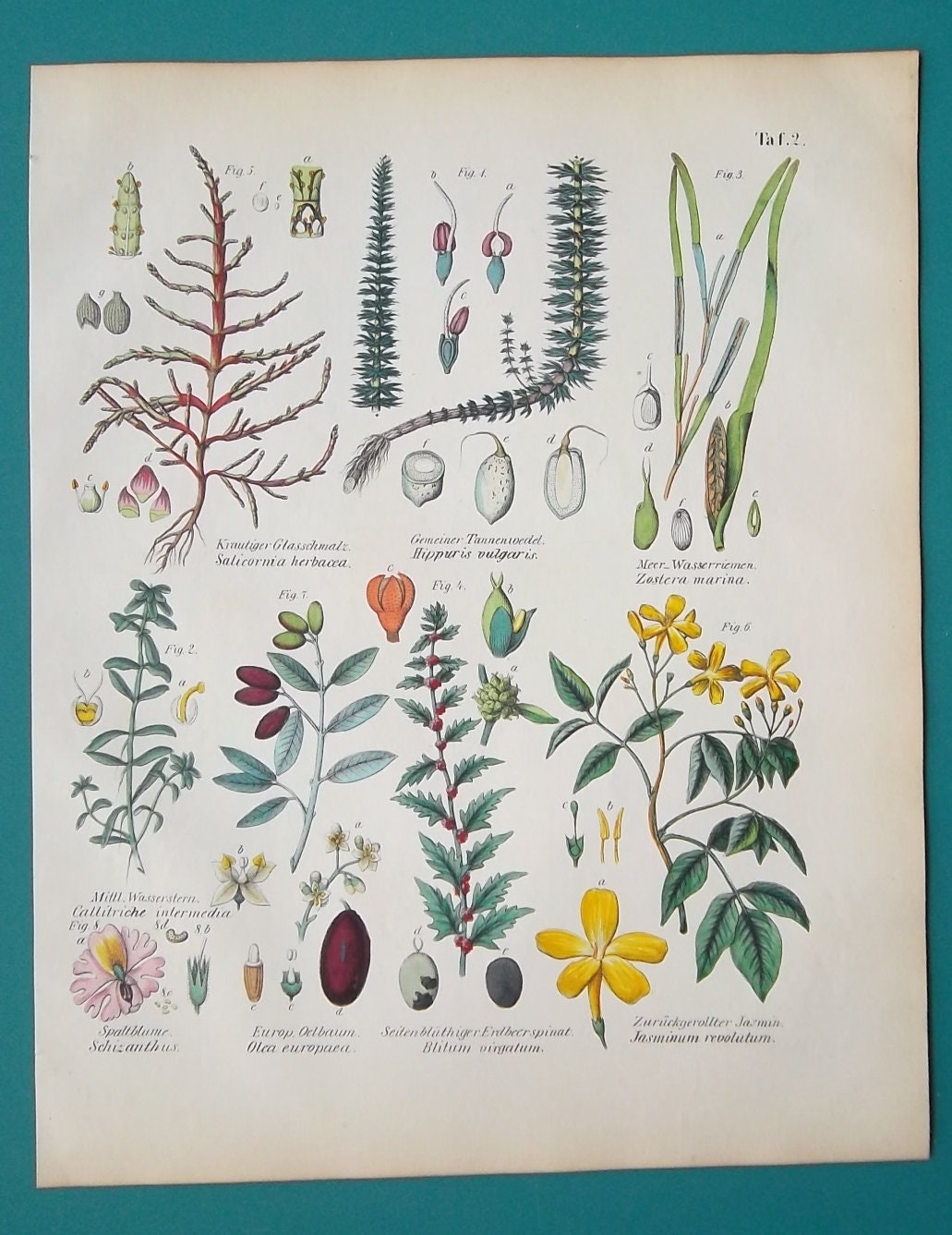This is a colored photograph of an antique, illustrated poster depicting various plants, seeds, and flowers. The poster, which appears to be from the mid-20th century based on its yellowed and worn edges, is placed on a dark green or teal background. The illustrations are created in a colored inline drawing style and are organized into two rows featuring a diverse array of plant species. The plants showcased range from green leaves and fern-like shapes to brown vines and flowering species with yellow blooms resembling buttercups and a distinct pink and yellow flower head. Each plant illustration is accompanied by its scientific Latin name and general information written in an old-fashioned, italicized script, difficult to read due to its small size. There are approximately 18 to 20 different designs displayed, each labeled sequentially as figure 1, 2, 3, etc., and they detail the progression of plant stages from seeds to mature plants. The overall scene captures the essence of an old scientific chart, possibly from a vintage book, highlighting the beauty and diversity of botanical life.